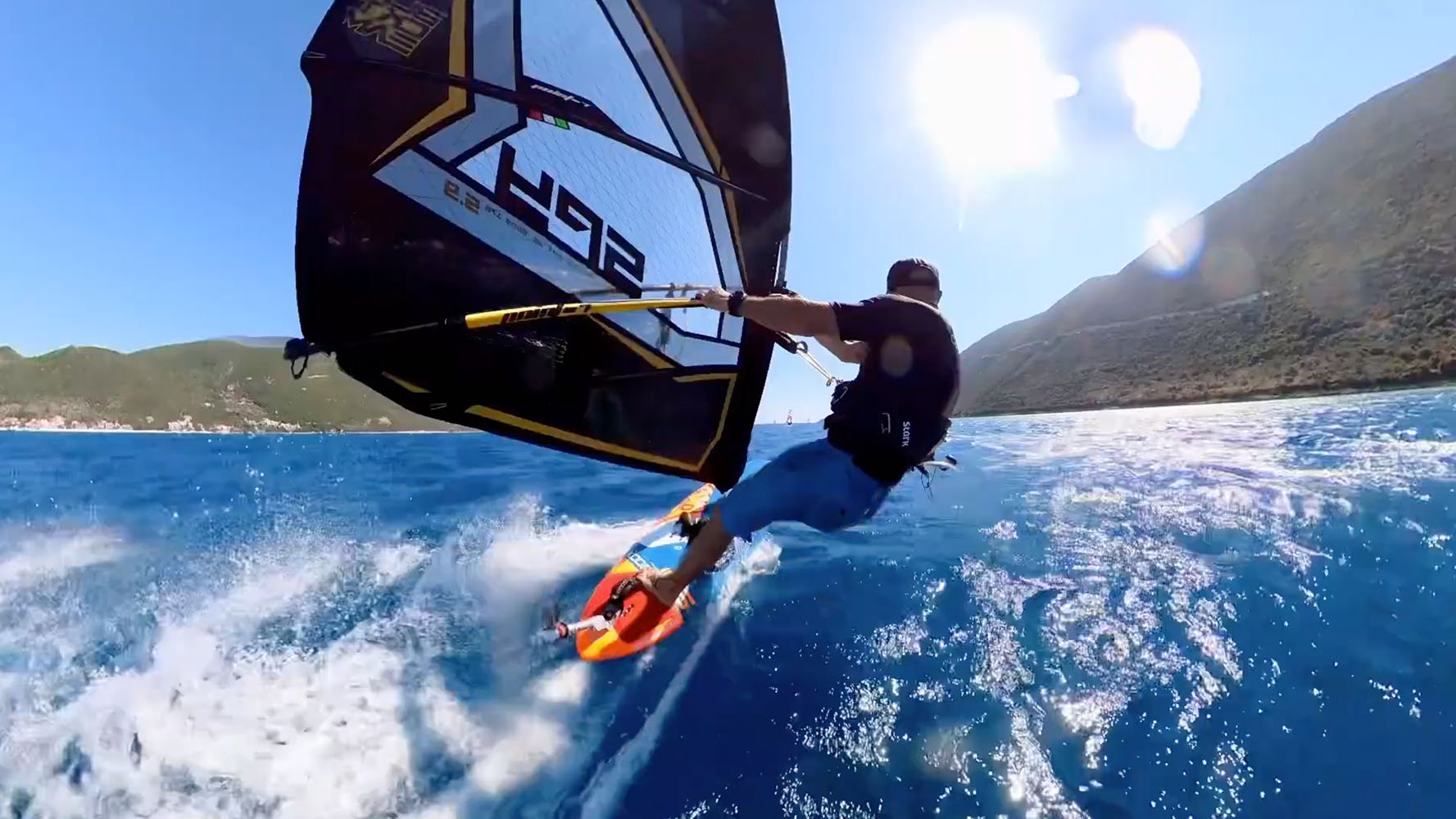In this dynamic and brightly captured photograph, likely taken from a GoPro on a selfie stick, we see a man windsurfing on the ocean on a sunny, cloudless day. The pristine, crisp blue water reflects the bright sunlight, and the presence of white spray trailing behind the windsurfer indicates a windy day, allowing for exhilarating speeds. The windsurfer is skillfully controlling his small craft, leaning into a turn with precision. His sail features the word "SPY" in reverse, with a clear middle section and dark blue around the edges, and his board is orange and blue. He is dressed in blue shorts and a black shirt, balancing on the windsurfing board between two islands or possibly within a channel, amidst green, lightly vegetated hills reminiscent of Southern California's scrubby landscapes. The scene is framed by sun rays and green hills on either side, adding depth to the vibrant, adventure-filled image.